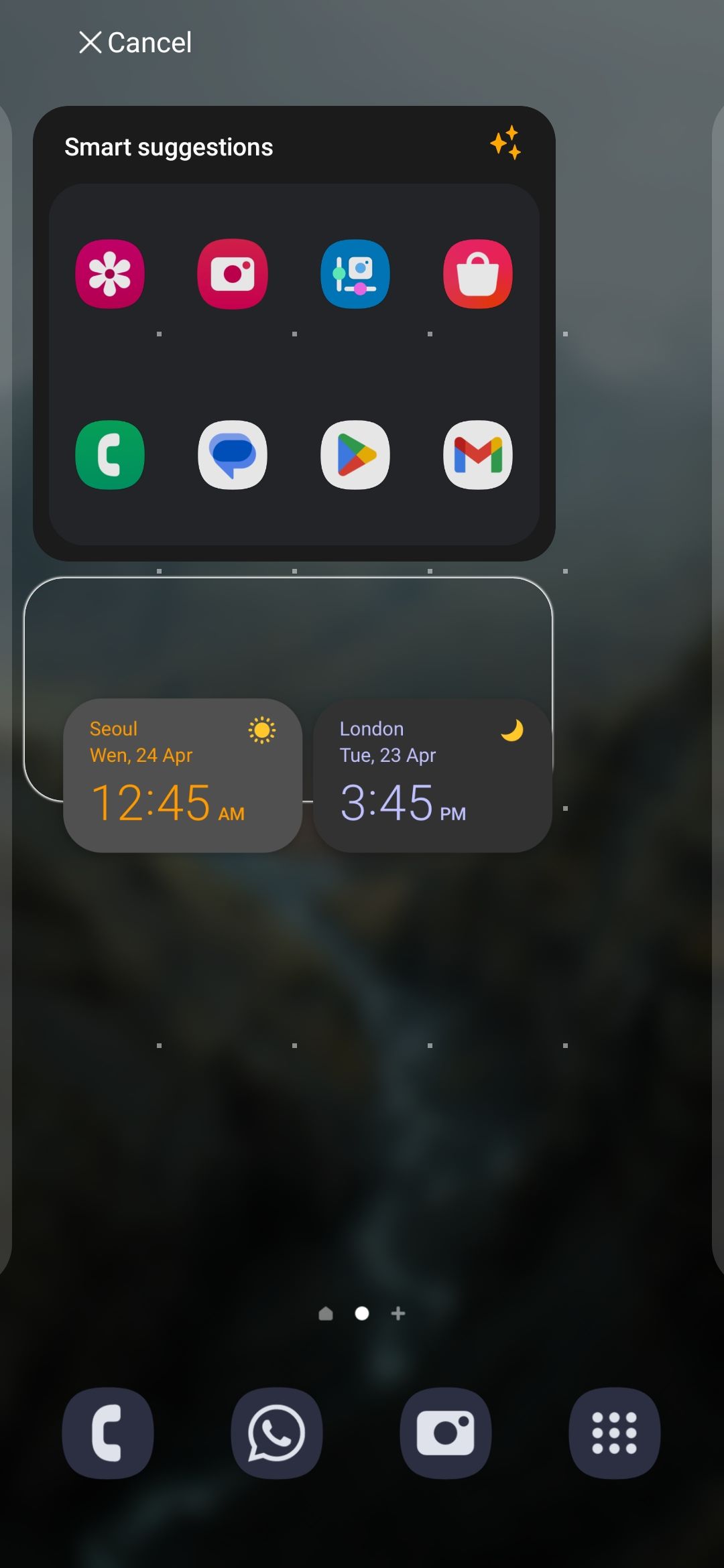This screenshot from a mobile phone showcases a background with a grey, abstract pattern reminiscent of paint swirling on water. At the top of the screen, a white "X" icon with the word "Cancel" appears in white font. Directly below this, a black translucent square features a black bar at the top with "Smart Suggestions" written in white lettering. In the right corner of this bar, three small golden four-pointed stars are displayed. 

Within the square, there are eight app icons arranged neatly. From left to right on the upper row: a pink icon with a white flower, a red icon with a white camera, a blue icon featuring a man standing by a computer in white, and a red icon with a white shopping bag. The lower row includes: a green icon with a white phone handset, a white icon with a blue chat bubble, a white icon with a rainbow arrow pointing to the right, and a white icon with a rainbow "M."

Beneath these icons is an empty rectangle containing two smaller rectangles that display the time and the weather.